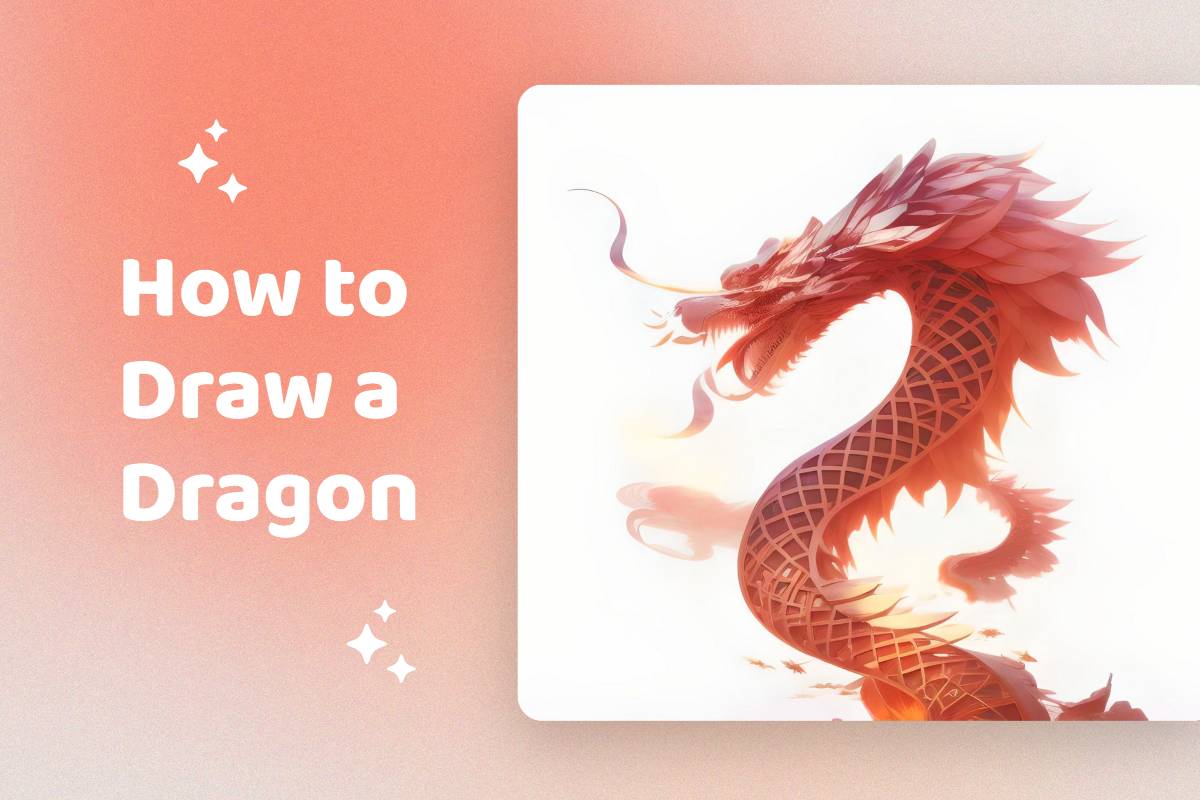The image is a horizontal, rectangular splash screen for a video tutorial titled "How to Draw a Dragon." The left side of the background features a diffuse orange watercolor wash that transitions to light beige at the bottom and dark gray to the right. Three white, four-pointed stars form a slight curve on the left, and the title "How to Draw a Dragon" is written in bold white capital letters, split into three lines. Further white stars are placed to the right of the word "Dragon."

The right side of the image contains a white rectangle inset into the background, housing a detailed illustration of a dragon. The dragon's head resembles a wolf with a heavy mane or feathers extending from the back and is positioned facing left. It has a serpentine, arched neck with visible dark red scales and gray tones, emitting fierce-looking white flames from its open mouth. The dragon's elongated body features dorsal fins and scales with cross-hatching, and the underbelly is black with red intersections. The overall appearance is fierce and ferocious, with watercolor splashes mimicking smoke or fire around it.